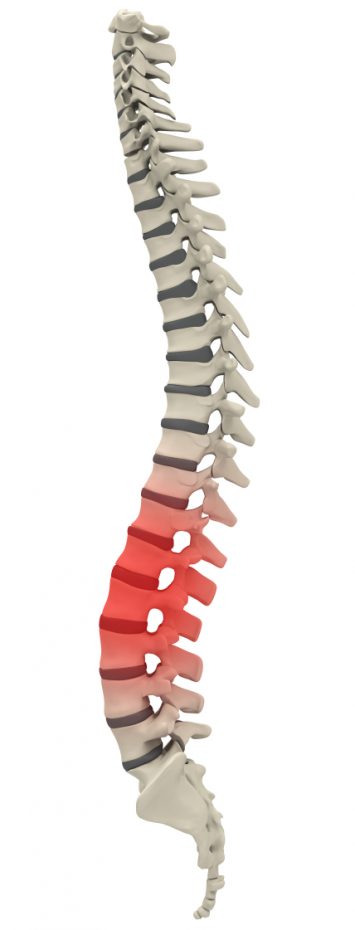This digital illustration depicts the human spine, highlighting both its anatomical structure and a specific region of concern. The top portion of the spine curves naturally to the right and then to the left, mimicking the inherent curvature found in a healthy spine. As the spine tapers down, it culminates in a pointed end resembling a tail.

The image accentuates a problematic area in the lower third of the spine, marked in red to indicate pain or inflammation. This reddish zone spans approximately four to five vertebrae, drawing attention to potential issues within that segment. Surrounding the highlighted area, the remaining sections of the spine are depicted in a natural bone-white color, with darker gray shading running through the center to represent the spinal cord.

Set against a clean, white background, this upright diagram effectively showcases the spine's overall shape and curvature, making it a useful tool for educational or diagnostic purposes.